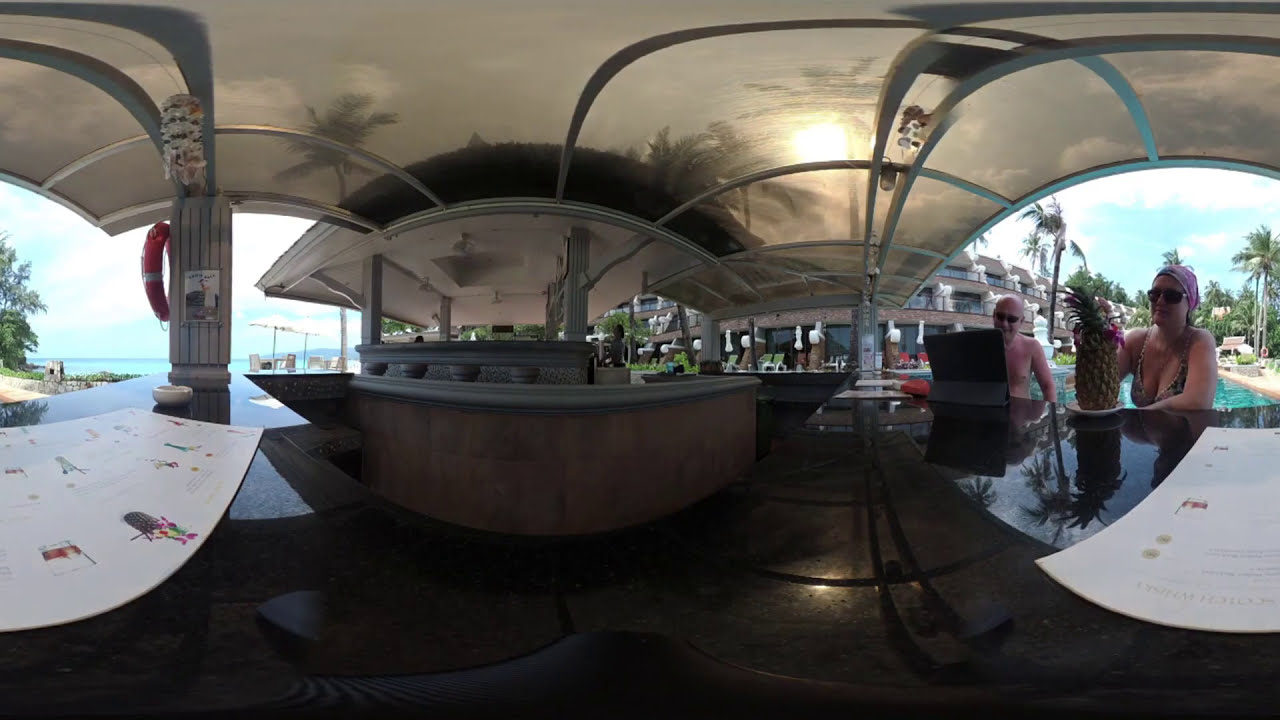This image captures a vibrant poolside bar scene, likely at a resort, featuring a central, bare counter made of brown marble. On the right side, there's a pool with people enjoying the water, while a building and tall palm trees frame the background against a bright, sunny sky. The bar has a gray, semi-transparent roof which allows the golden setting sun and distant trees to be visible through it. 

Notably, two patrons are present at another part of the bar: a shirtless man interacting with a large screen, possibly ordering from a menu, and a woman in sunglasses, a pink swim cap or bandana, and a bikini top. She has a large pineapple drink in front of her. White drink menus with pictures are displayed on either side of the bar. The entire scene evokes a lively, tropical vacation vibe with people relaxing and indulging in drinks.